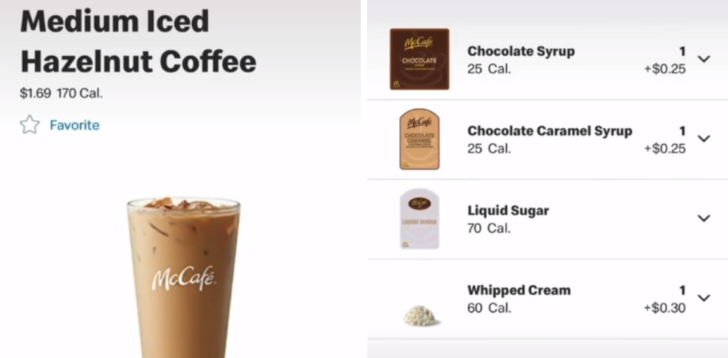The image is a split-screen snapshot of the McDonald's app, showcasing a product and its customizable options. 

On the left side, the app features the details of a "Medium Iced Hazelnut Coffee" in black font against a whitish-gray background. The product name is prominently displayed at the top. Just below it, the price is listed as $1.69, also in black font, and to the right, the calorie count is indicated as 170 calories. Below this information, a blue star icon accompanied by the word "Favorite" highlights the option to favorite this item. At the bottom center of this section, there is an image of a glass with the McCafe logo in white font, showing the glass filled with iced hazelnut coffee.

On the right side, the image presents various customization options for the coffee, allowing users to enhance their drink with different syrups, sugars, and whipped cream. The available options are "Chocolate Syrup," "Chocolate Caramel Syrup," "Liquid Sugar," and "Whipped Cream." Each option is detailed with the additional calorie count listed below the name. To the left of each name, there is a small image of the corresponding syrup, sugar, or whipped cream. To the right, the quantity and the additional cost for each add-on are provided, offering users a convenient way to personalize their coffee.